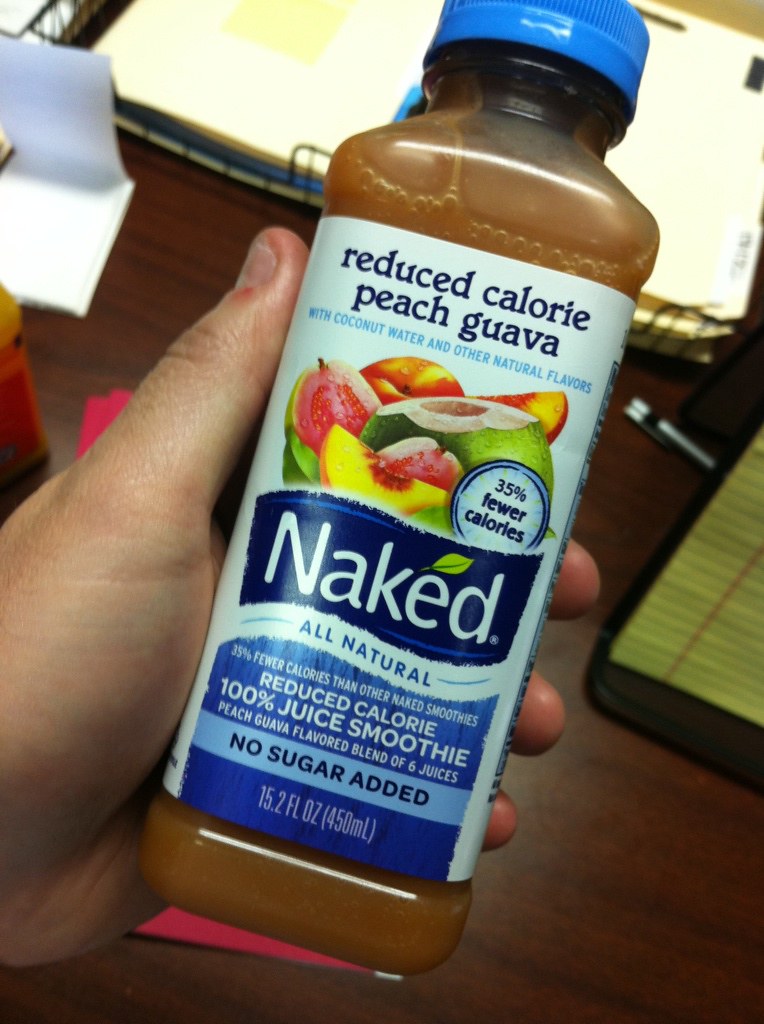A close-up image captures a Caucasian hand holding a bottle of Naked-branded reduced calorie peach guava juice smoothie. The bottle, featuring vibrant illustrations of peaches and pears, is cradled in the left hand, coming in from the lower left-hand side of the frame. The label highlights that it contains 100% juice with no sugar added, and boasts 33% fewer calories. The light brown juice inside is capped with a distinct blue lid. The hand holding the bottle shows signs of nail-biting, with sparse fingernails and some redness under one of them. The background reveals a dark wooden desk, topped with a brown clipboard holding a yellow notepad in the upper right corner, which adds context to the setting. The bottle is 15.2 fluid ounces in size and includes coconut water and other natural flavors, emphasizing its refreshing qualities.